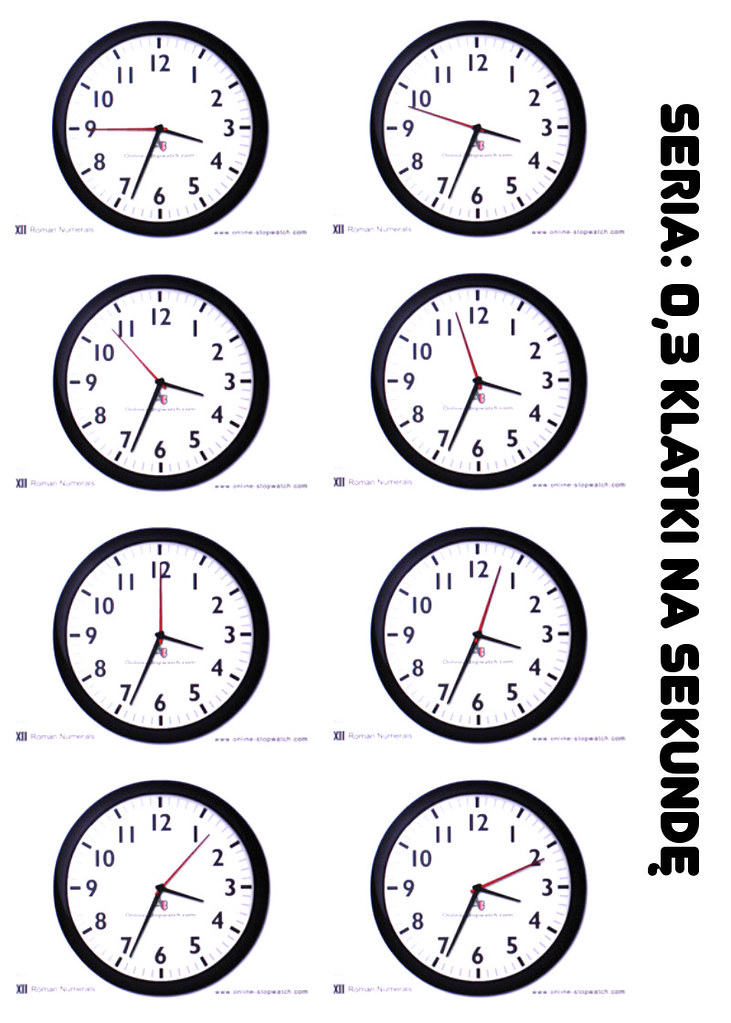This image is a poster-style arrangement featuring eight clocks displayed against a white background. Each clock has a consistent design: a round, black plastic frame enclosing a white clock face, marked with black numbers from 1 to 12 and black dash marks for the minutes. The clocks also feature a short black hour hand, a long black minute hand, and a single red second hand. The clocks are arranged in four rows of two, resulting in a neat vertical formation of paired clocks.

Beneath each clock, there is small black text that is too tiny to be legible. Notably, the times shown on the clocks vary, with some displaying the same time while others diverge. On the right side of the poster, bold block letters spell out "S E R I A . . 0 , 3 K L A T K I N A S E K U N D E." This phrase, alongside the uniform yet slightly varying times on the clocks, suggests an abstract or conceptual art piece, possibly pertaining to different moments in time or a study of second intervals.